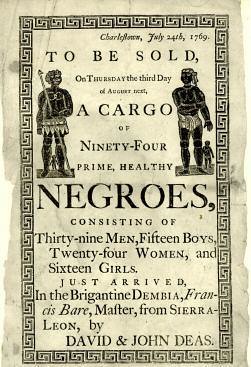The image shows an old, wrinkled, and faded piece of paper resembling an antique newspaper or flyer, dated July 24th, 1769, likely from Charleston. The document, surrounded by black and white designs, announces the sale of slaves and reads: "To be sold on Thursday, the 3rd day of August, a cargo of 94 prime healthy negroes, consisting of 39 men, 15 boys, 24 women, and 16 girls, just arrived in the brigantine Dambia, Francis Bear, Master, from Sierra Leone by David and John Deas." The disturbing details and presence of images of African American individuals underline the grim history of slavery in the country.